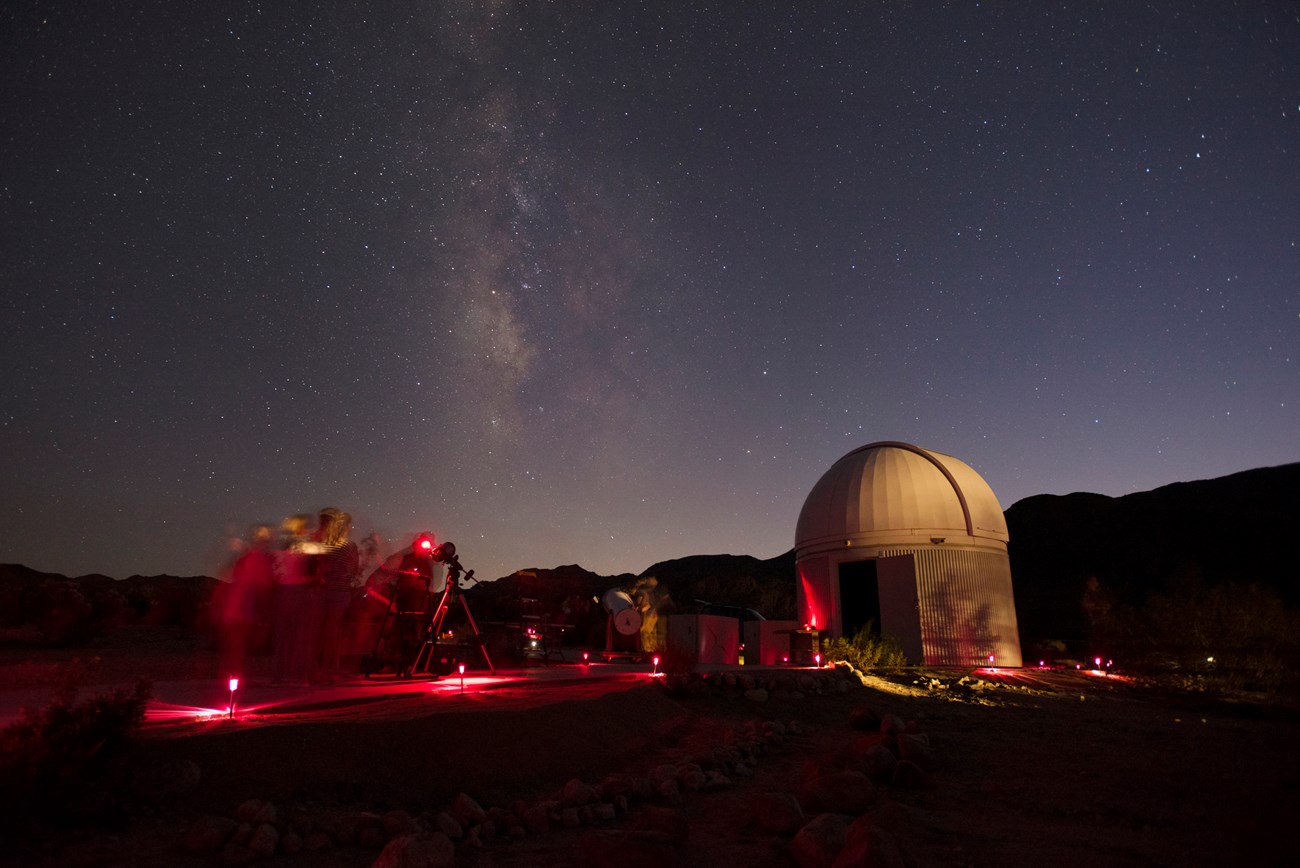The image is a full-color, square, outdoor scene taken at night with artificial lighting. The top two-thirds of the photo showcase a starry night sky with visible stars and the center of the Milky Way. The image is slightly blurry, adding a dreamy quality to the scene. Slight mist or smoke can be seen in the air, enhancing the atmospheric effect. Towards the bottom right, there's a white domed building, likely an observatory for a telescope, resembling a small planetarium with a gold-colored, circular top. In the center left, there is a platform adorned with red lights and several blurred individuals who appear to be gazing through a smaller telescope at the sky. Tall hills are visible in the background, bridging the sky and the platform scene below. The red lights create a striking contrast against the night, reinforcing the observatory's purpose and adding to the intricate details of the overall image.